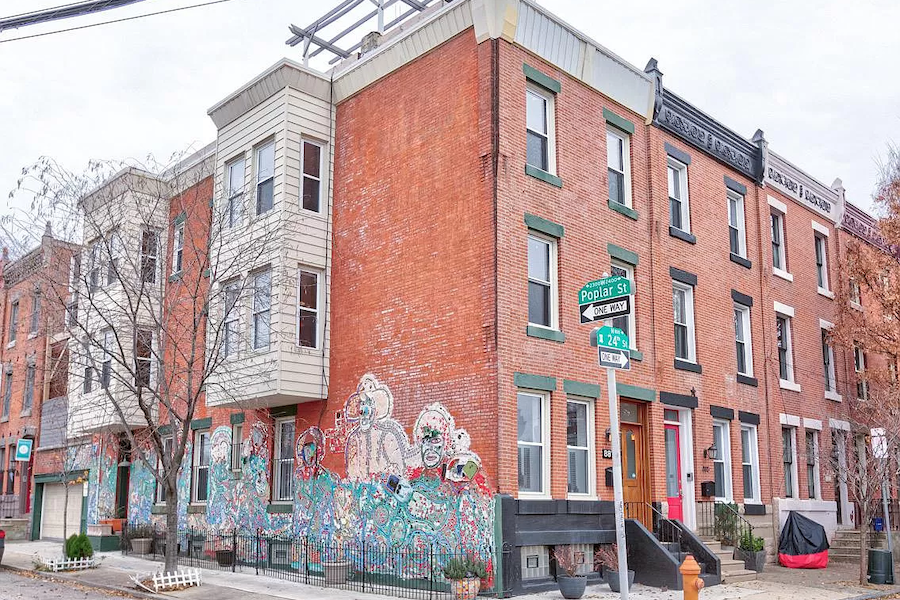The image captures a corner view of an older apartment complex or townhouse located at the intersection of Poplar Street and 24th Street, with both streets designated as one-way. The three-story building, constructed from brownish-red brick, features several units, each with approximately six two-pane windows. On the right side of the building, short sets of stairs lead up to the entrances of at least the first-floor apartments. The left side of the building is adorned with a mural depicting people, though the artwork appears weathered and is fading, with the lower halves of the figures painted in vibrant colors. Additionally, white window panes protrude from the side of the building, adding to its distinct appearance. The overall state of the structure, with signs of age and wear, suggests it is situated in an older, possibly less affluent area of the city.